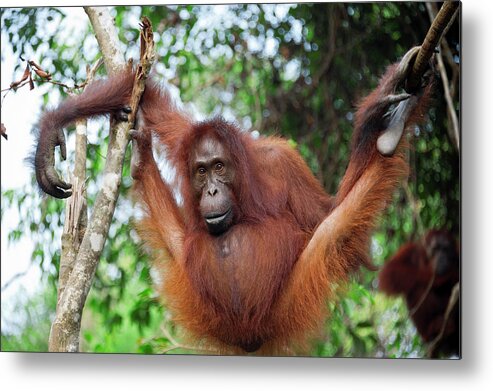This detailed photograph features an orangutan suspended between two trees, displaying its impressive agility. The orangutan's right arm and right foot are gripping the same branch, with its elbow hooked and its toes wrapped securely around the limb. Simultaneously, its left arm and left foot are gripping another branch on the opposite side, giving it a sprawled appearance with legs widely spread. The orangutan's bright orange fur contrasts with its long, gray face and notably large hands. Its arms, noticeably longer than its legs, showcase its powerful build. The orangutan's round belly adds to its distinct look. It gazes directly at the camera with an almost intense, curious expression. The background is lush and vibrant, filled with dense green jungle foliage. Patches of cloudy sky with glimpses of blue peek through the trees on the upper left side. Additionally, a second orangutan, similar in appearance, is visible in the lower right part of the image, hanging from the trees. This companion adds depth to the scene, enhancing the sense of a thriving jungle habitat.